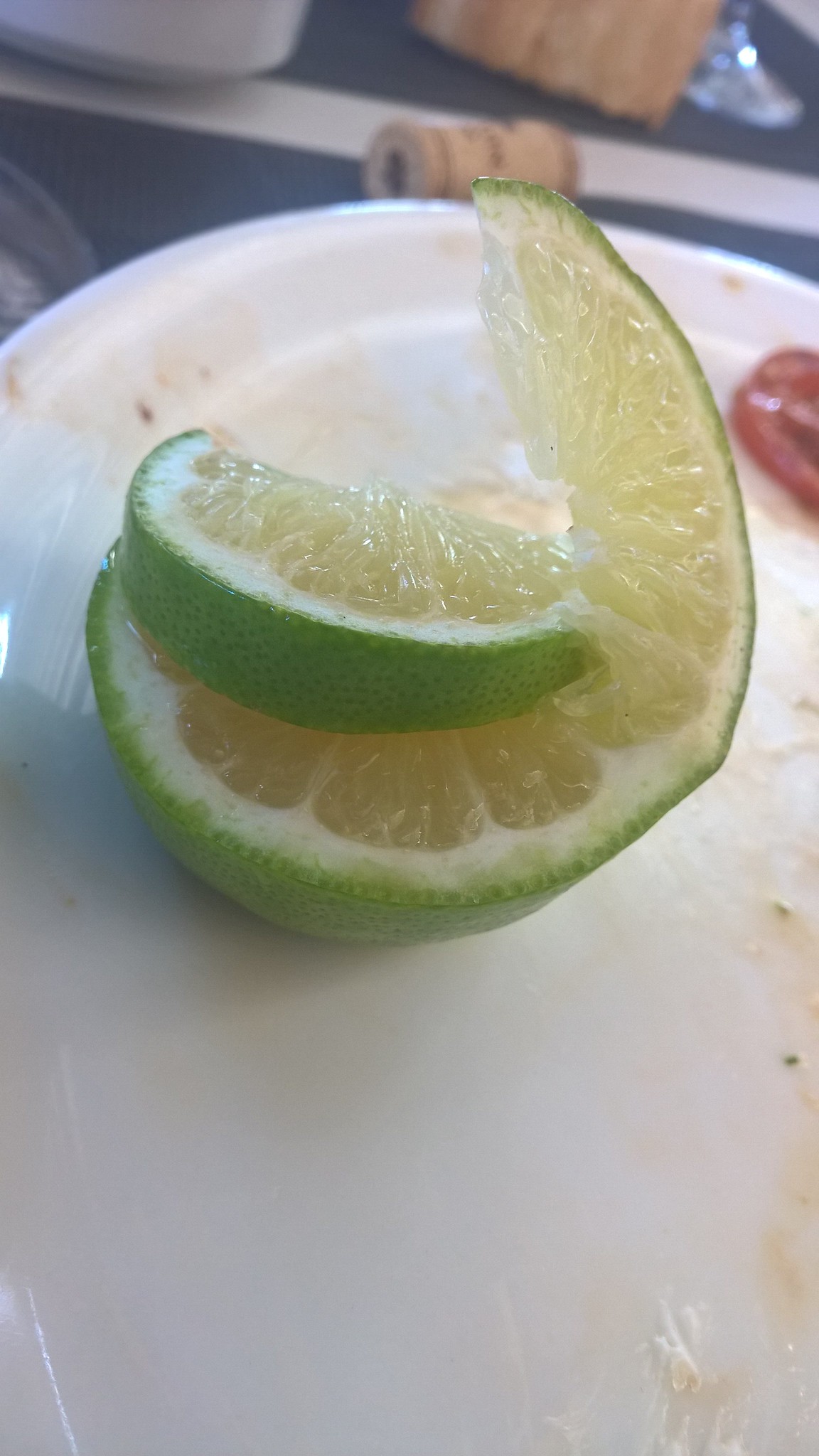The image depicts a close-up of a sliced lime resting on a slightly messy white plate, likely in a restaurant or dining room setting. The lime has been halved, with one half propped upright and slightly folded over itself, displaying both the vibrant green rind and the juicy yellow interior. The plate beneath the lime is speckled with seeds and lime juice, suggesting recent food preparation. In the background, which is out of focus, there are hints of a dining environment: a brown wine cork, a blue and white striped tablecloth, the base of a wine glass, and what appears to be a tilted spice container. The overall scene captures the vivid detail of the lime and the subtle context of a dining or prep area beyond.